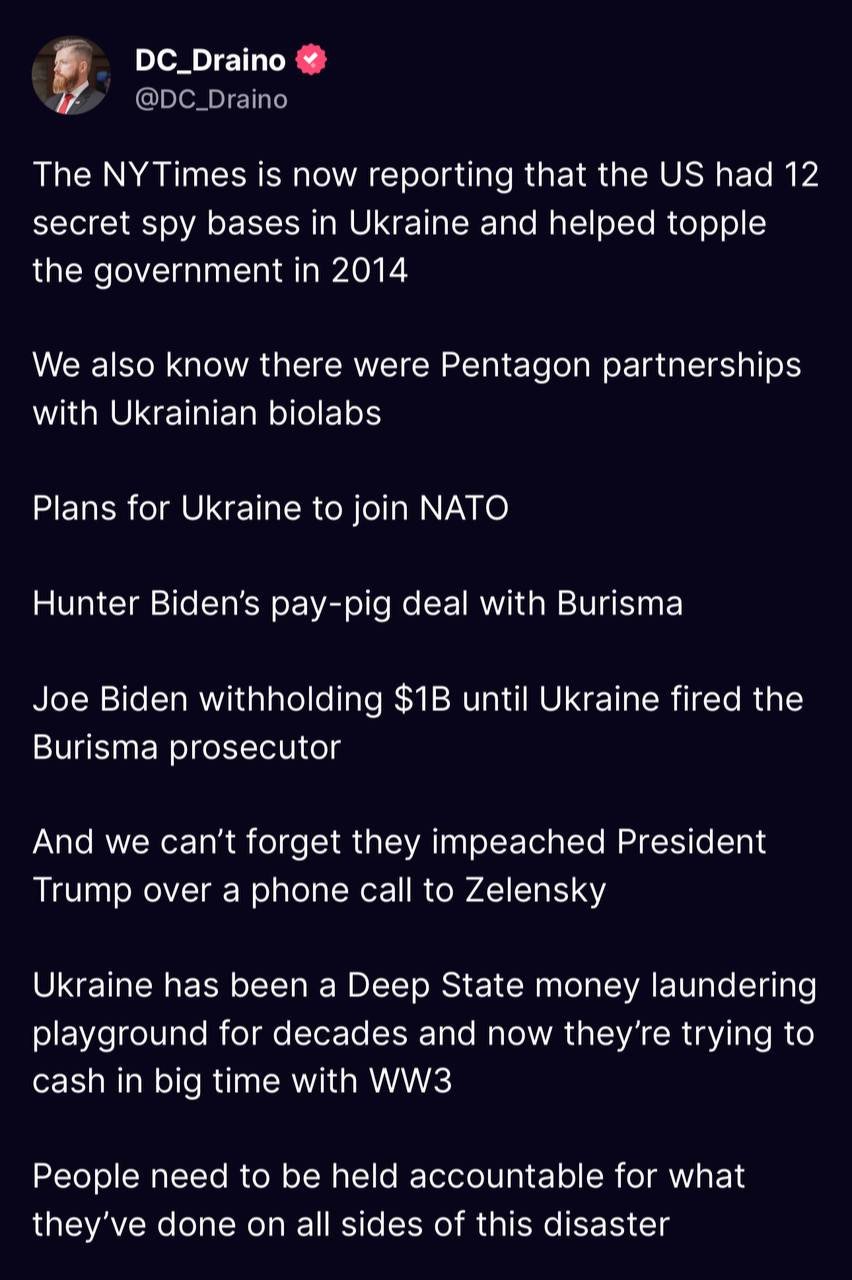**Screenshot of a Twitter Post by @DC_Draino**

The image is a screenshot of a Twitter post from the user @DC_Draino, distinguished by a red circle with a white check mark beside the profile image. The profile picture shows a person in a sharp suit and red tie, facing left.

Caption:
*The New York Times is now reporting that the U.S. had 12 secret spy bases in Ukraine and helped cobble the government in 2014. We also know that there were Pentagon partnerships with Ukrainian bio labs. Plans for Ukraine to join NATO. Hunter Biden’s big deal with Burisma. Joe Biden withholding $1 billion until Ukraine fired the Burisma prosecutor. And we can’t forget they impeached President Trump over a phone call to Zelensky. Ukraine has been a deep state money laundering playground for decades and now they’re trying to cash in big time with World War III. People need to be held accountable for what they’ve done on all sides of this disaster.*

The background of the post is either black or a very dark blue, making the white text stand out prominently.